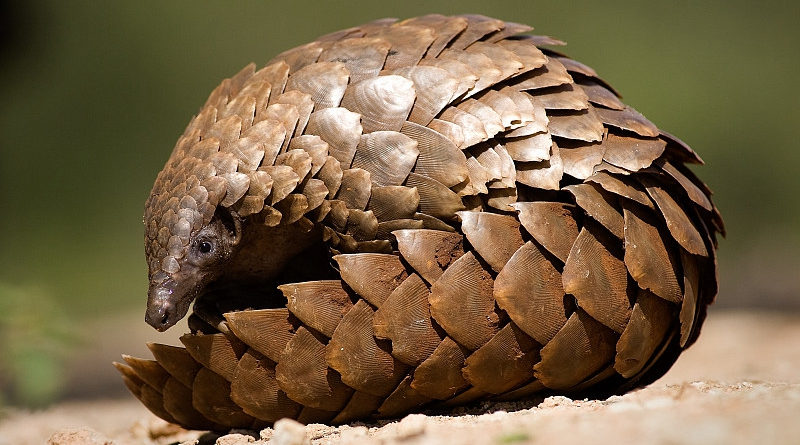This photo features a small brown pangolin, an unfamiliar yet fascinating animal that resembles a prehistoric creature or an armadillo. The pangolin's body is entirely covered in layers of shiny, brown scales that extend from its sharp, pointy face down to its long tail. Its tiny eyes and wooden, armor-like scales give it a somewhat daunting appearance. The pangolin is curled up into a ball, obscuring any view of its limbs and conveying a sense of it closing itself off from the world. It rests on light tan or brown dirt, with a blurred background suggesting dark green leaves and trees. The overall scene captures the pangolin's unique, almost otherworldly presence.